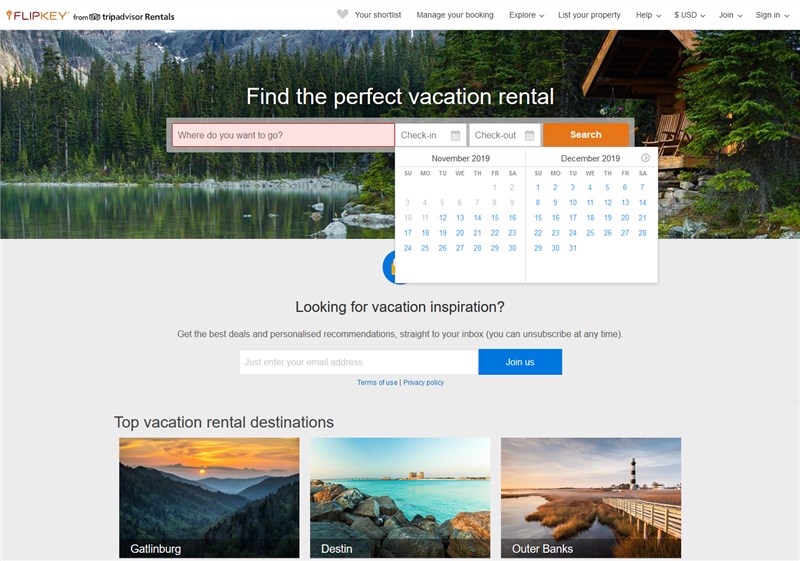The image appears to be a screenshot of a vacation rental website called FlipKey, which is affiliated with TripAdvisor Rentals. The top left corner features the FlipKey logo, while to its right, the text reads "From TripAdvisor Rentals." Across the top right section of the image, there are various navigation categories starting with "Sign In," followed by "Join," "USD," "Help," "List Your Property," "Explore," "Manage Your Booking," "Your Shortlist," and finally, a heart icon.

In the top center, the text "Find the Perfect Vacation Rental" is prominently displayed in white. Directly below this headline are several search boxes. The first box prompts users with the question, "Where do you want to go?" To its right are two smaller boxes for selecting check-in and check-out dates, both featuring a small calendar icon. The last box is labeled "Search" in white text on an orange background.

Underneath these search boxes, two calendars are visible, one for November 2018 on the left and another for December 2018 on the right. Further down, a message in the middle of the image reads, "Looking for vacation inspiration? Get the best deals and personalized recommendations straight to your inbox. You can unsubscribe at any time."

This detailed layout suggests an interface designed to facilitate the search for vacation rentals, with user-friendly navigation and clear prompts to enhance the booking experience.